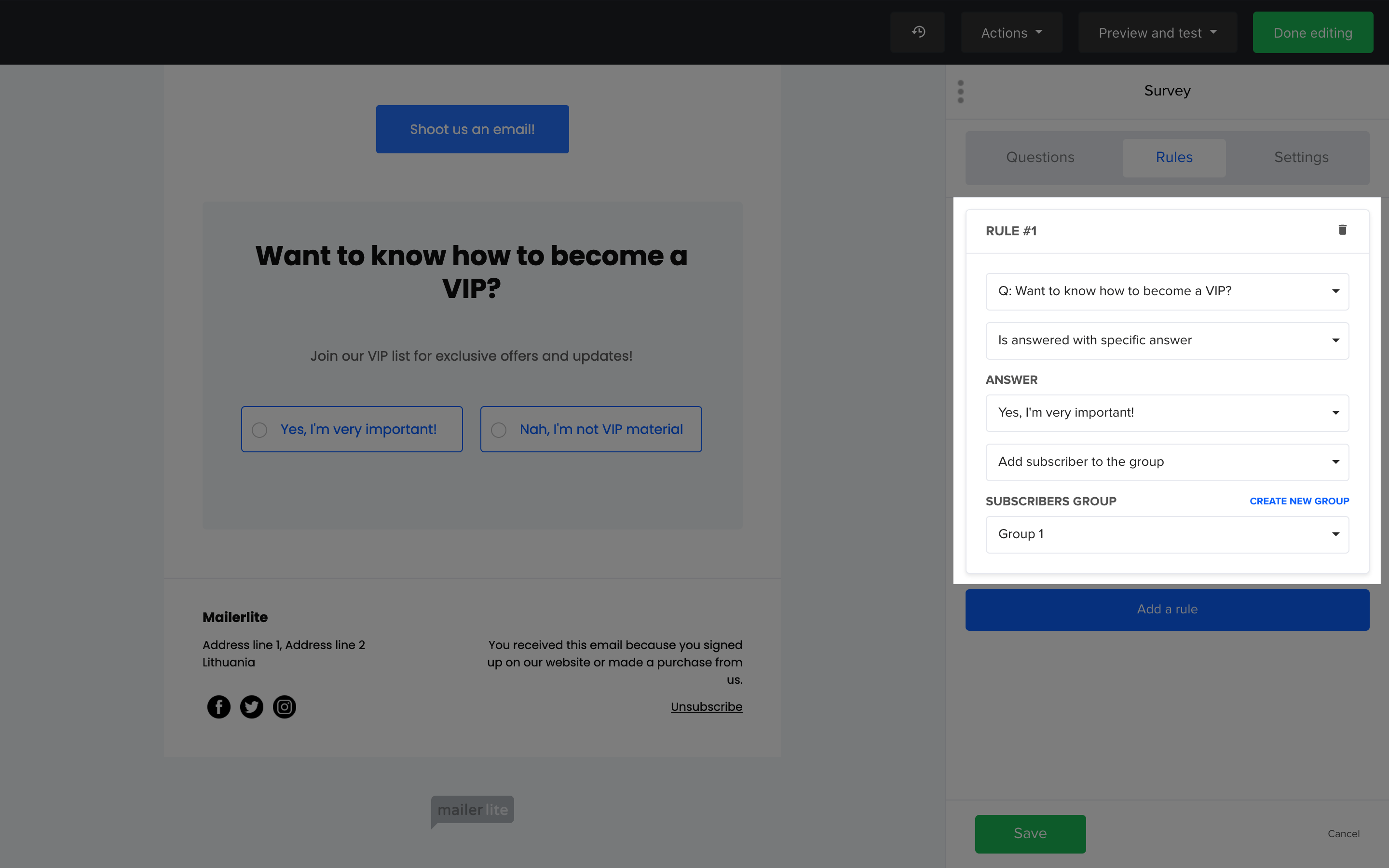This image is a screenshot from a webpage featuring a grayish background with a prominent white pop-up box designed to capture the viewer's attention. On the right side of the box, the bold title "Rule Number One" is displayed, followed by an icon of a trash can at the end of the same row. Below this title, there are two interactive rectangles, each containing a dropdown menu. 

The first rectangle poses the question, "Want to know how to become a VIP?" and offers dropdown options for answers. The first answer states in all uppercase black letters, "YES! I'M VERY IMPORTANT!" with an exclamation point. The second dropdown option underneath reads "Add subscriber to your group."

Beneath these options, another section contains a dropdown menu labeled "Subscriber Group," with an option to "Create New Group" highlighted in blue text alongside it. Additionally, there is an existing group option labeled "Group One" with its own dropdown menu.

In the muted background, various blue links can be seen, one of which invites users to "Shoot us an email." Another section reiterates the VIP inquiry, presenting the options "Yes, I'm very important" and "Nah, I'm not VIP material."

Overall, the layout is crafted to guide users through the VIP subscription process while offering clear call-to-actions within an accessible and organized interface.